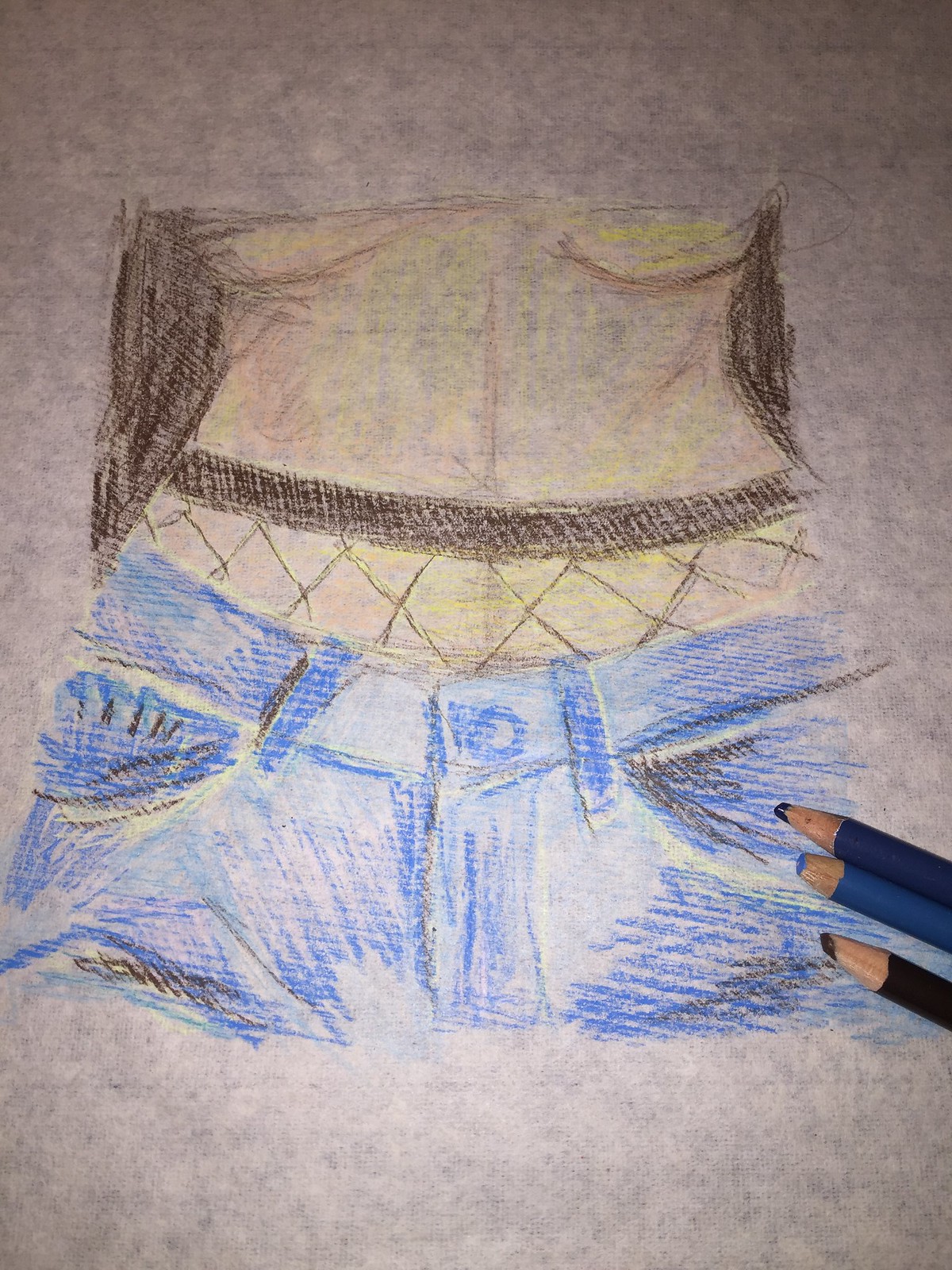This is a highly detailed colored pencil drawing created on darkly shaded paper. The artwork captures a woman's figure from just below her breasts to the top of her groin. She is wearing cut-off blue jean shorts with visible pockets, paired with what appears to be fishnet underwear, showcasing a striking fishnet pattern. The woman's hands or arms seem to be positioned behind her back, and she has long brown hair flowing down. The curvature of her breasts is subtly suggested at the top, but without any explicit anatomical details such as nipples. Overall, it's a reasonably well-executed drawing, demonstrating a good command of colored pencils.